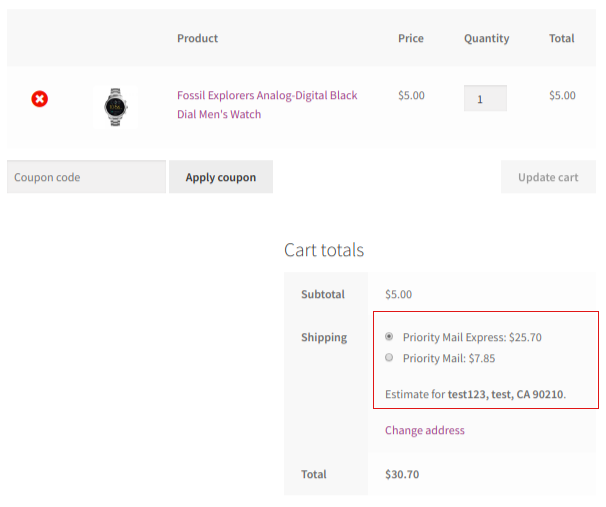This image appears to be a composite of two screenshots depicting an online shopping cart interface. 

In the upper section of the image:

- The first row features a gray background with the headers: Product, Price, Quantity, and Total.
- The second row has a white background, displaying a red "X" for item removal, a picture of a watch, and a purple hyperlink titled "Fossil Explorer's Analog-Digital Black Dial Men's Watch," indicating it has been clicked. 
- Under the Price column, the watch is listed at $5.
- The Quantity column displays a fill-in box with the number 1 selected.
- The Total column reflects the price of $5.

Further down:

- There is a section to enter a coupon code, accompanied by a gray button with black bold font labeled "Apply Coupon."
- To the right, there is another gray button in dark gray font, labeled "Update Cart." The various gray shades make readability challenging.

In the lower section of the image:
 
- There is a "Cart Totals" area with a gray background:
  - Subtotal is listed as $5.
  - The Shipping section provides options for "Priority Mail Express" or "Priority Mail," with "Priority Mail Express" ($25.70) selected and highlighted in a red border. 
  - An estimated shipping address is indicated as "Test, 123 Test, CA 90210."
  - A "Change Address" option is available via a purple hyperlink.

- The overall Total is calculated to be $30.70.

This detailed breakdown provides a comprehensive understanding of the shopping cart's interface and its elements.